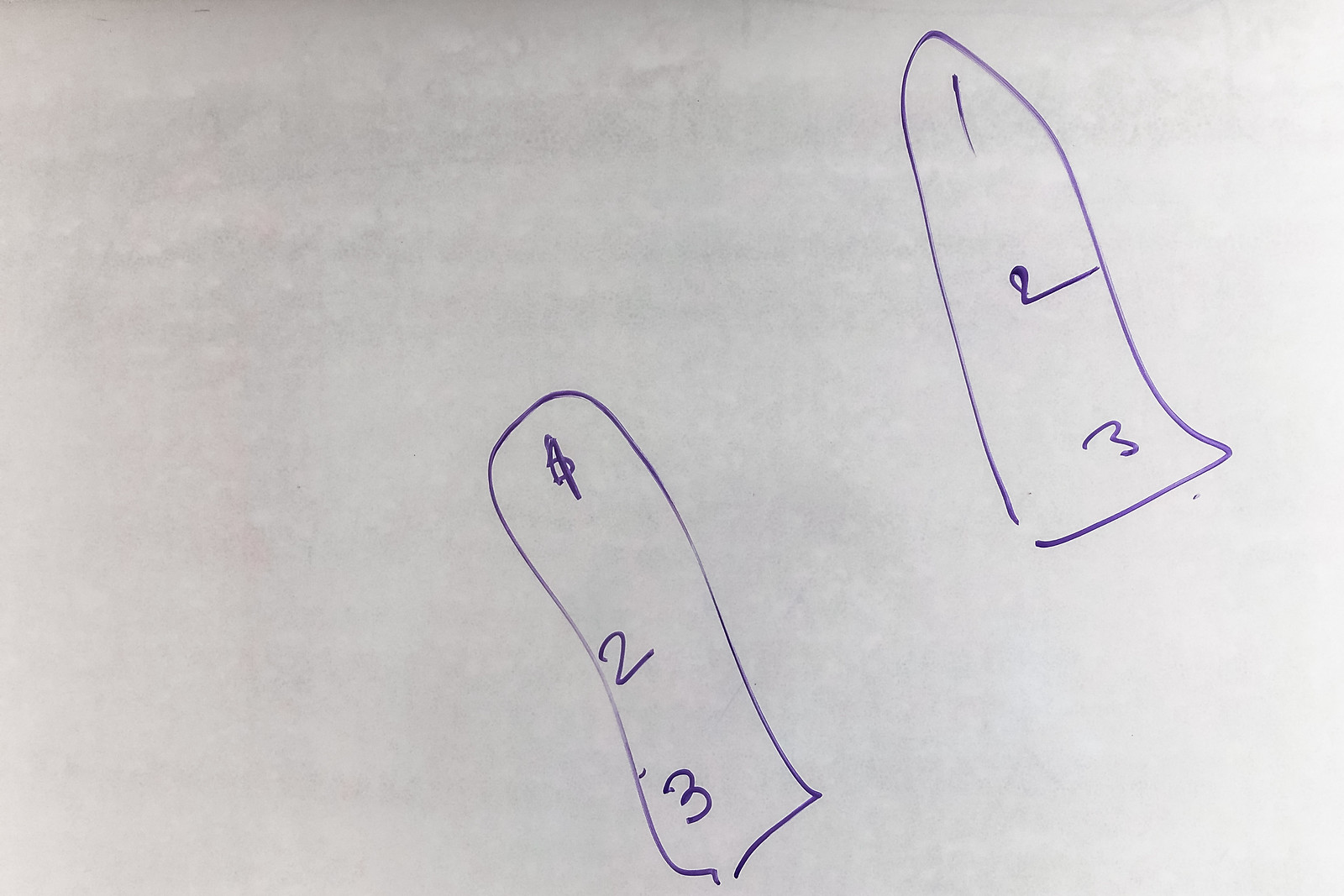A piece of white paper with a soft gray hue, created by subtle shading along the top, is depicted in the image. This shading accentuates barely visible white splotches, particularly noticeable within the gray area. 

Centrally positioned and extending towards the bottom of the paper, there is an illustration drawn with a thin purple or blue marker. The drawing features a cylindrical shape which starts from the bottom, curves upwards and around to the right, then descends diagonally to the left. At the top of this first cylinder is the number "4." Approximately two inches below the "4" and about an inch and a half further down, there is another cylindrical shape. This second cylinder, unlike the first, has a more squared-off top.

At the top-middle section of the second cylinder, there is a hastily drawn line indicating the number "1." Beneath this is a "2," with the back line of the number extending far to the right. Below that, there is a "3." The numbers appear to be written hastily, suggesting that the person who drew them was in a hurry.